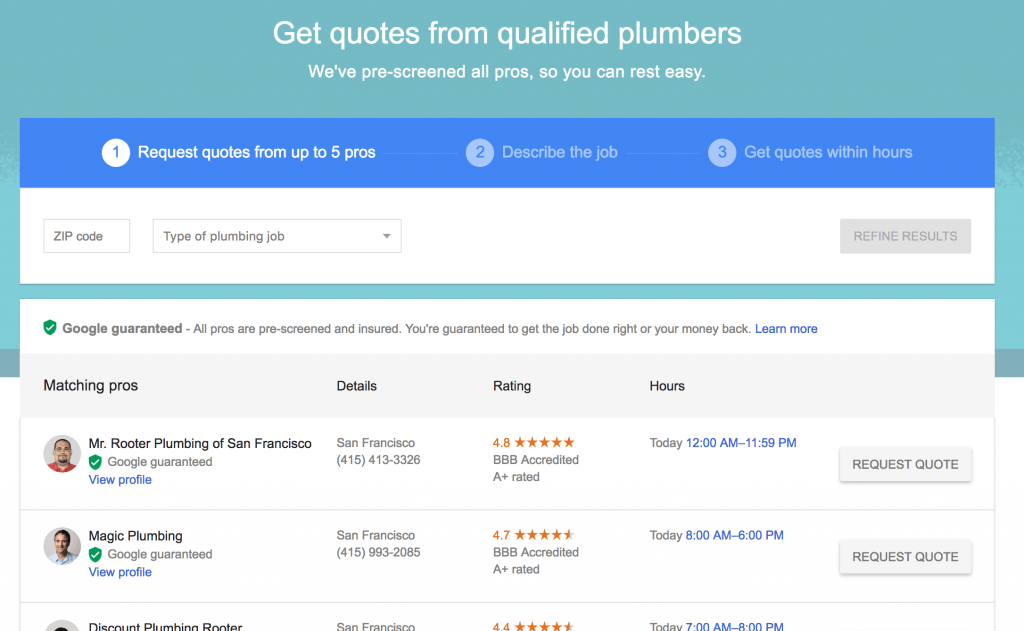Screenshot of a Plumbing Quote Comparison Website

This screenshot captures a vibrant blue, white, and teal website designed to provide users with multiple quotes from qualified plumbers. At the very top of the page, a prominent header reads: "Get quotes from qualified plumbers. We've pre-screened all pros so you can rest easy." 

The process to obtain quotes is outlined in three simple steps:
1. **Request quotes from up to five pros.**
2. **Describe the job.**
3. **Get quotes within hours.**

A user-friendly interface is provided, featuring a field to input the user's zip code, a drop-down menu to select the type of plumbing job needed, and a button to refine the search results.

Below the main search area, a certification statement reads, "Google Guaranteed. All pros are pre-screened and insured. You're guaranteed to get the job done right or your money back," alongside a "Learn More" button for additional information.

The section labeled "Matching Pros" displays profiles of available plumbers. The first two visible profiles are:

1. **Mr. Ruder Plumbing of San Francisco**: Includes a small profile picture of a man, accompanied by detailed information about the plumbing service.
2. **Magic Plumbing**: Noted as Google Guaranteed, with clickable "View Profile" and "Request Quote" buttons beside their details.

The third profile is partially visible. Each plumber's listing includes their rating, operating hours, and a button at the end to request a quote, ensuring transparency and ease of contact for users seeking reliable plumbing services.